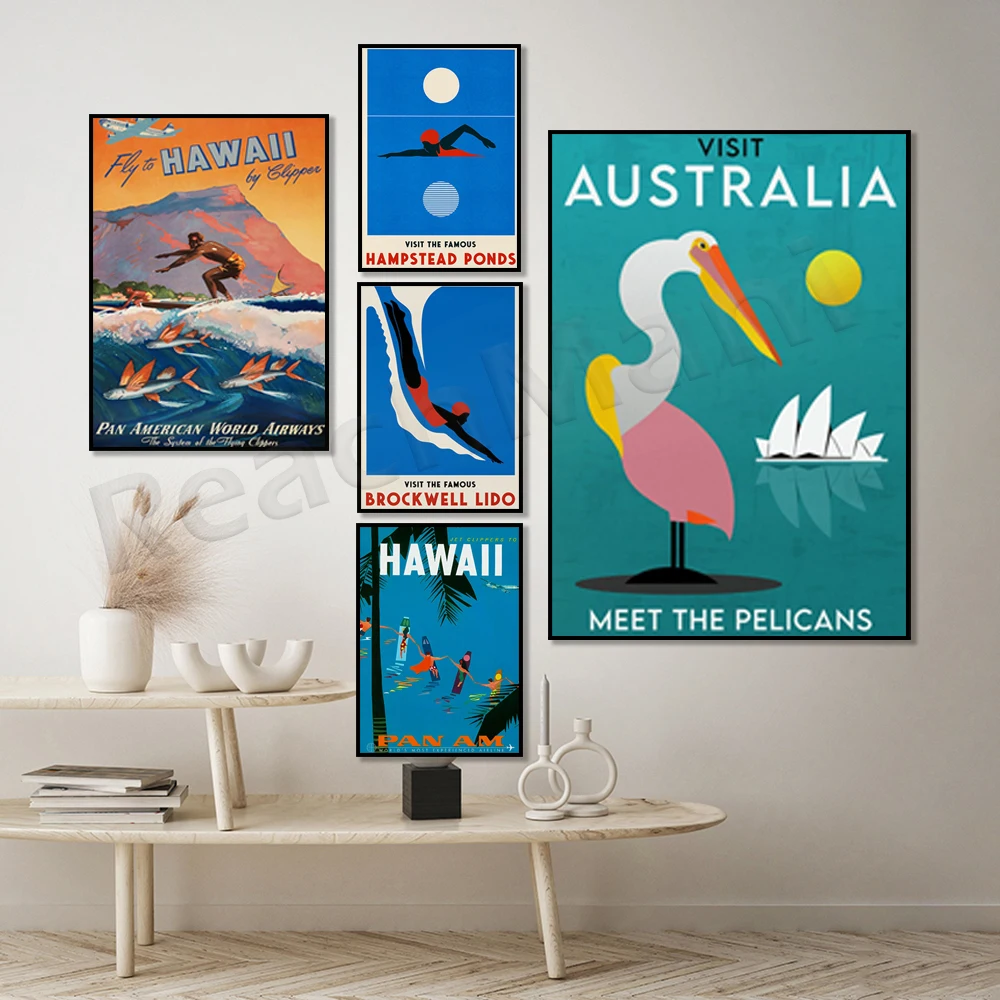In this vertical image, a white wall serves as the backdrop for several vibrant posters advertising travel destinations. The posters include titles such as "Visit Australia, Meet the Pelicans" featuring a pelican and a sun, "Fly to Hawaii, Pan American World Airways" with an image of someone surfing, and others labeled "Hampstead Palms," "Brockwell Lido," and another "Hawaii" poster. The wall art features illustrations of surfers, swimmers, and pelicans. Below the posters, a white table is neatly arranged with various knick-knacks: white vases, some with plants, a stack of books, U-shaped decorative objects, rings, and what appears to be a speaker. The entire setup rests on a floor adorned with a white and striped brown rug.